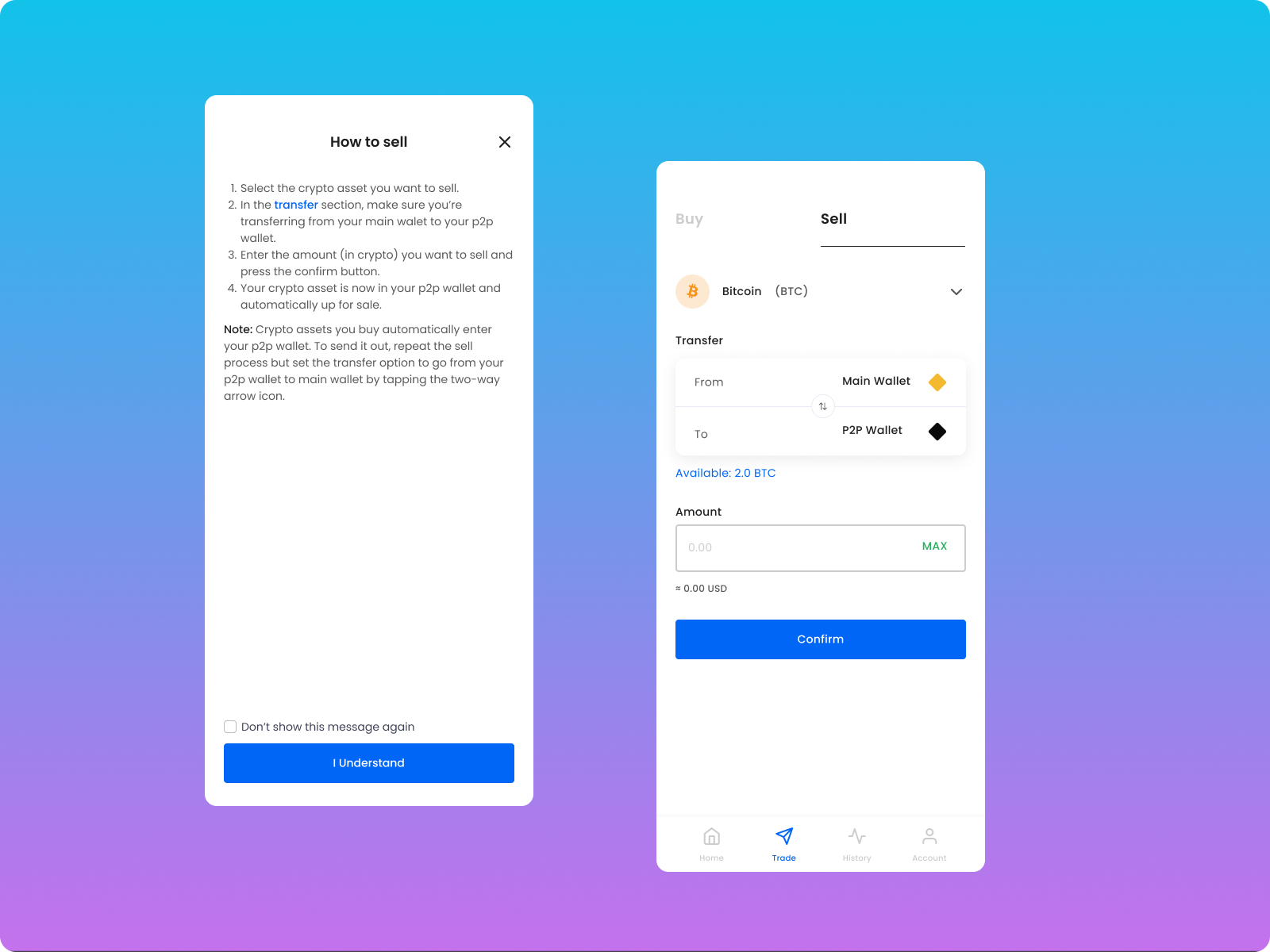This image features a collage of two instructional screenshots related to Bitcoin or cryptocurrency transactions, displayed within a square frame with rounded edges. The photo has a gradient background, transitioning from light blue at the top to a light violet at the bottom, with a darker middle section where the blue fades into purple.

Situated on the left side of the image, the first screenshot displays a guide titled "How to Sell" in black font. Below the title, a series of instructions detail the steps needed to sell a crypto asset:
1. Select the crypto asset you want to sell.
2. In the transfer section, ensure you are transferring from your main wallet to your P2P wallet.
3. Enter the amount in crypto.
4. Your crypto asset is now in your P2P wallet and automatically up for sale.
At the bottom of this screenshot, there is a note followed by a blue "I understand" message box and a checkmark option to "Don't show this again."

On the right side, a second screenshot illustrates a transaction page with a "Buy" and "Sell" header. The "Sell" option is highlighted with black text and an underline. Bitcoin is selected, and instructions reiterate transferring from the main wallet to the P2P wallet. The main wallet is represented by an orange diamond icon, while the P2P wallet is signified by a black diamond. Beneath these details is a blue "Confirm" button in white font.

The overall visual presentation, combined with the detailed instructional content, offers a clear guide for users engaging in cryptocurrency transactions.